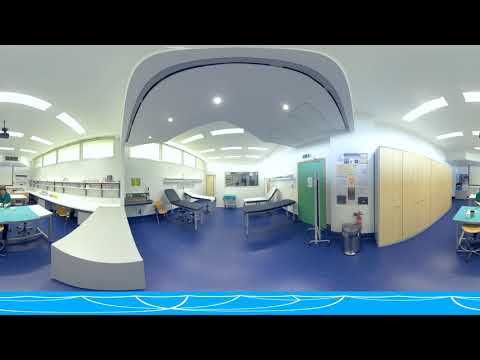The image depicts a horizontally aligned, computer-generated panorama of a modern, advanced medical facility or lab. The scene is brightly lit with rectangular fluorescent lights in the white ceiling, enhancing the visibility of the entire space. The walls are white, adorned with windows at the top and containing various furniture and equipment. 

In the center, there are four examination tables, two on each side of the room. The back two tables are white, while the front two are dark gray, designed with adjustable backs for patient comfort. Flanking these tables on the left and right are black tables and counters, equipped with stools underneath and possible lab equipment situated behind them. 

The flooring is a blend of light gray and dark blue tiles, and a blue strip with white swirled lines runs just above the thick black border at the bottom of the image. Additional features include a set of large green doors, a trash can next to the door area, and closed closets or cubbies along the right side wall. The room also contains some beige-colored furniture and shelves with unidentified equipment, contributing to an overall sterile yet advanced ambiance.